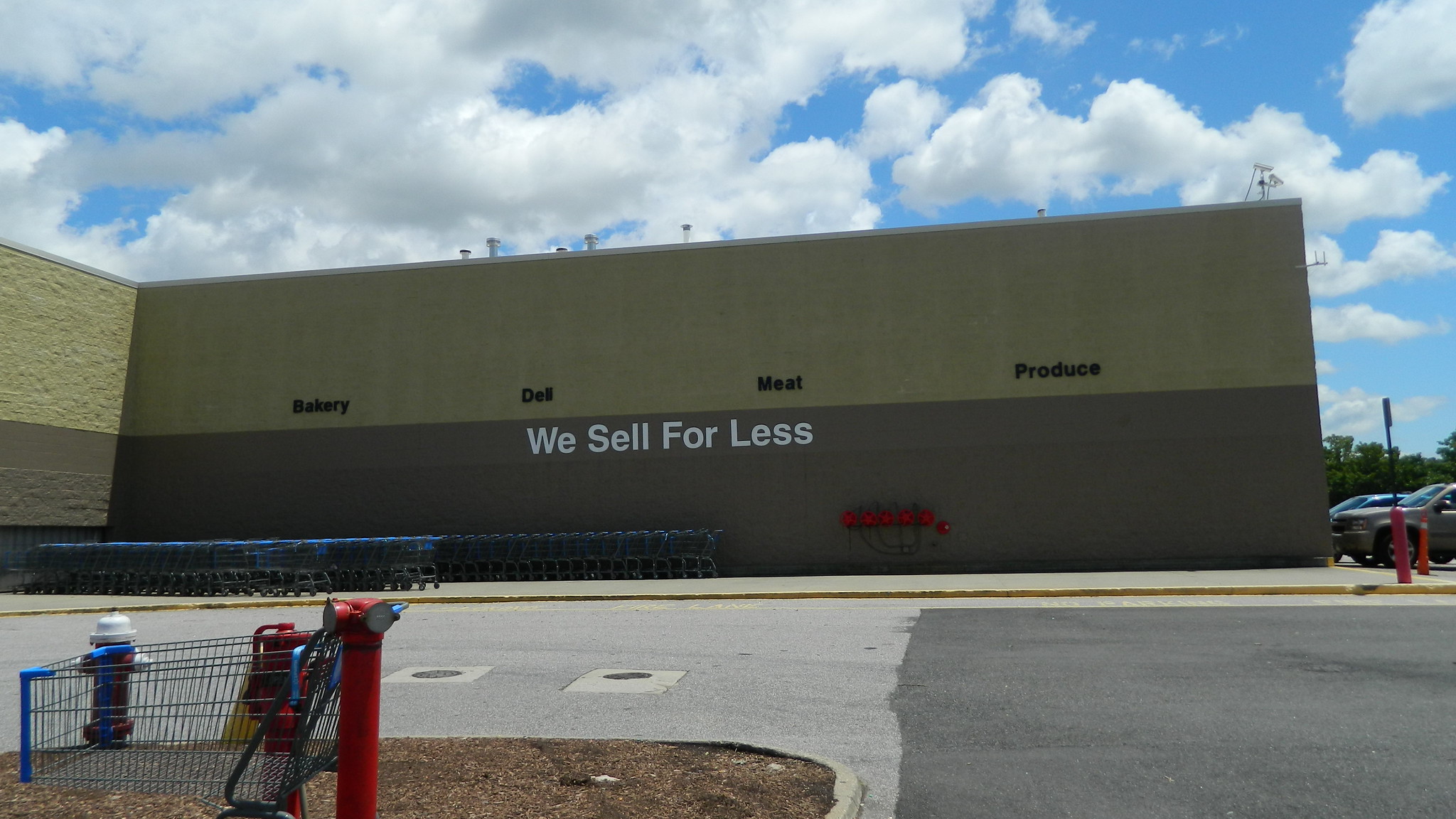This daytime photograph captures the exterior of what appears to be a Walmart store. The image prominently displays the side of the building, marked with black lettering indicating the departments: "Bakery," "Deli," "Meat," and "Produce." Below these department names, a slogan in white letters reads, "We Sell for Less." In front of the store, rows of blue-handled shopping carts are neatly organized. The scene also shows part of the parking lot and a street. To the left corner at the bottom of the frame, there is a small curb area with exposed dirt, a fire hydrant, and a lone shopping cart parked beside a red post.